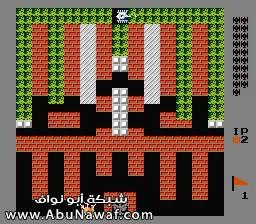This image is a screenshot of an 80s-style video game showcasing a classic, pixelated aesthetic. The game screen is framed with a gray border forming a rectangular shape. At the bottom left corner, there’s some Arabic text above a URL that reads "www.abunawaf.com." The game’s layout features a series of horizontal and vertical brick paths, mimicking tunnels and pathways. The lower section has a mix of red bricks and black areas, transitioning to green areas representing foliage as you move upward. In between the paths are gray and white spaces which could signify different structures or barriers. Near the center, the player's character appears among these structures. At the top right portion, within a gray area, there are various symbols including a flag marked with the number 1 and IP2 above it, possibly indicating a score or player identifier. Additionally, there are numerous small icons that resemble spaceships or lives remaining. The overall design and elements evoke the feel of classic gaming systems, like Atari or Sega, emphasizing chunky graphics and simplistic detail.